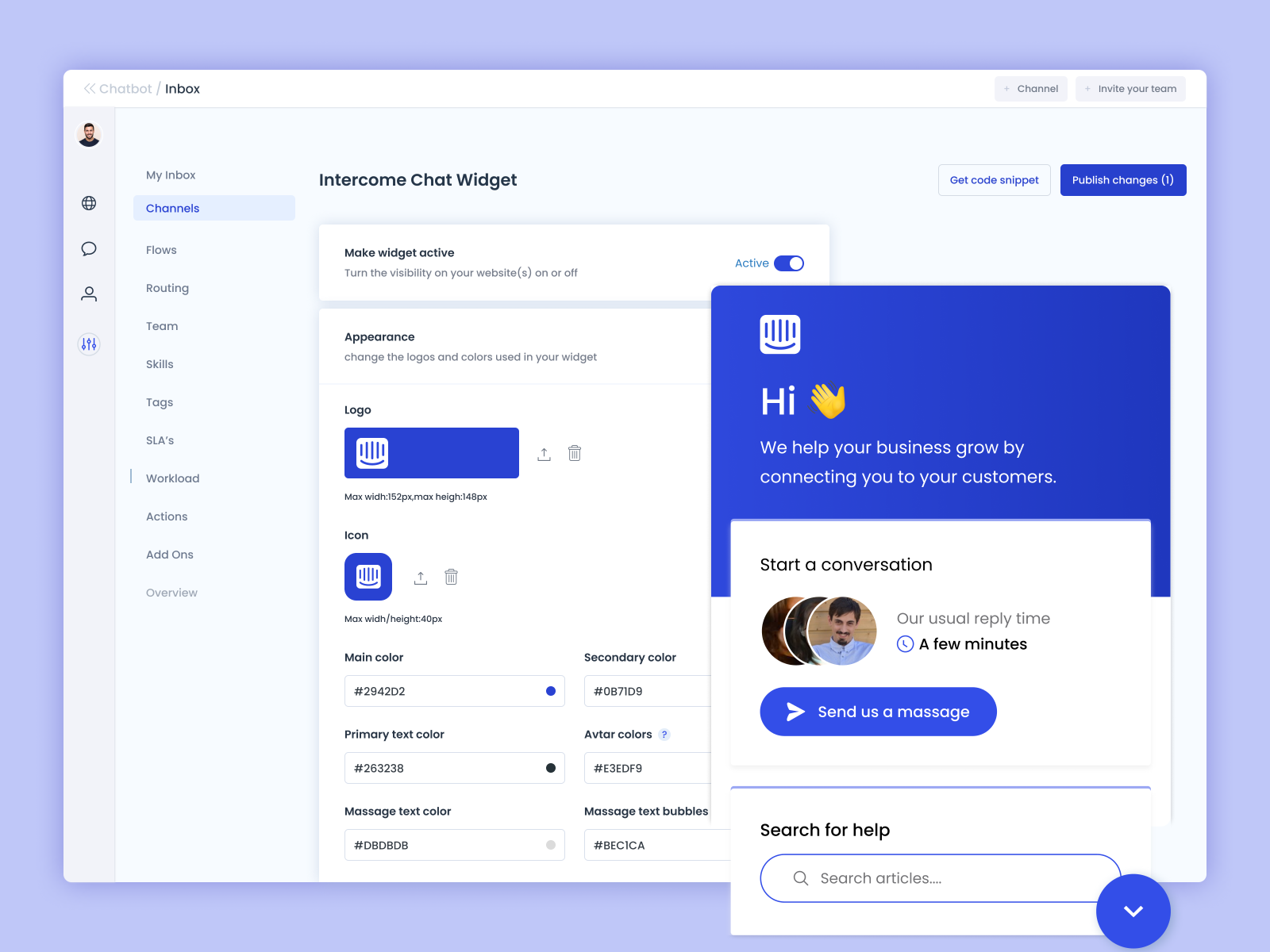Screenshot Description:

The image captures a detailed view of a user interface with various menu items and options. The primary background is light blue. Centrally, there's a screenshot with a white bar at the top featuring gray, double left-hand arrows, followed by the text "chatbot /" in gray and "inbox" in black. On the right-hand side of this bar are three gray boxes with drop-down arrows. The first box is labeled "channel," the second "plus channel," and the third "plus invite your team."

Below this, a light blue line stretches horizontally across the screen. Adjacent to this, on the far left, is a small vertical gray bar with an emoji depicting a man. Directly beneath this are four icons arranged vertically: a globe icon, a chat icon, a profile/account icon, and an icon featuring a sliding bar, with this last icon appearing selected.

The left-hand menu lists several options in black text. The selected item, indicated by a blue highlight, is "channels." Other entries include "my inbox," "flows," "routing," "team," "skills," "tags," "SLAs," "workload," "actions," "add-ons," and "overview." A vertical line beside these items suggests multiple selections.

To the right of this menu, in bold black text, are the words "intercom chat," followed by "intercom chat widget." Below this is a white box containing the bolded text "make widget active," with regular black text underneath stating, "turn the visibility on your website(s) on or off." There is also a blue link labeled "active" and a blue toggle switch.

A larger white section below this is labeled "appearance." It includes gray text explaining, "change the logos and colors used in your widget." The section features a black label "logo" with a blue bar underneath. Inside the blue bar is a white icon with five vertical lines of varying heights and an arc beneath it. To the right are upload and trash icons. The maximum dimensions are listed as "152px width" and "148px height."

Similarly, under "icon," a blue square displays the same icon, with upload and trash icons to its right and a maximum size of "40px x 40px." Further descriptions include "main color" with a gray outline box containing "#2942d2" and a blue dot, "primary text color" with a gray outline box containing "#263238" and a black dot, and "message text color" with "#dbdbdb" and a light gray dot.

Additionally, to the right of "main color" is "secondary color" with "#0871d9." Under "avatar colors," a light blue circle with a darker blue question mark is shown. The box beneath contains "#e3edf9," followed by "message text bubbles" with "#becica." To the right is a blue rectangular box with the same icon and the word "hi" in white text. Below this is a hand-waving image and the message, "We help your business grow by connecting you to your customers."

Overlapping the bottom of this blue box is a white box saying "start a conversation" in black text, accompanied by three overlapping avatars. The top avatar depicts a man with a mustache and a beard on his chin. The text next to it, "Our usual reply time," is followed by a blue circle with a phone icon, stating "a few minutes." There is also a blue oval with a white right-hand arrow and the text "send us a message."

At the bottom of the screen is a blue line, "search for help" in black text, and a blue outlined oval with the text "search articles" accompanied by a magnifying glass icon. Finally, a dark blue circle with a white drop-down arrow rounds out the interface.